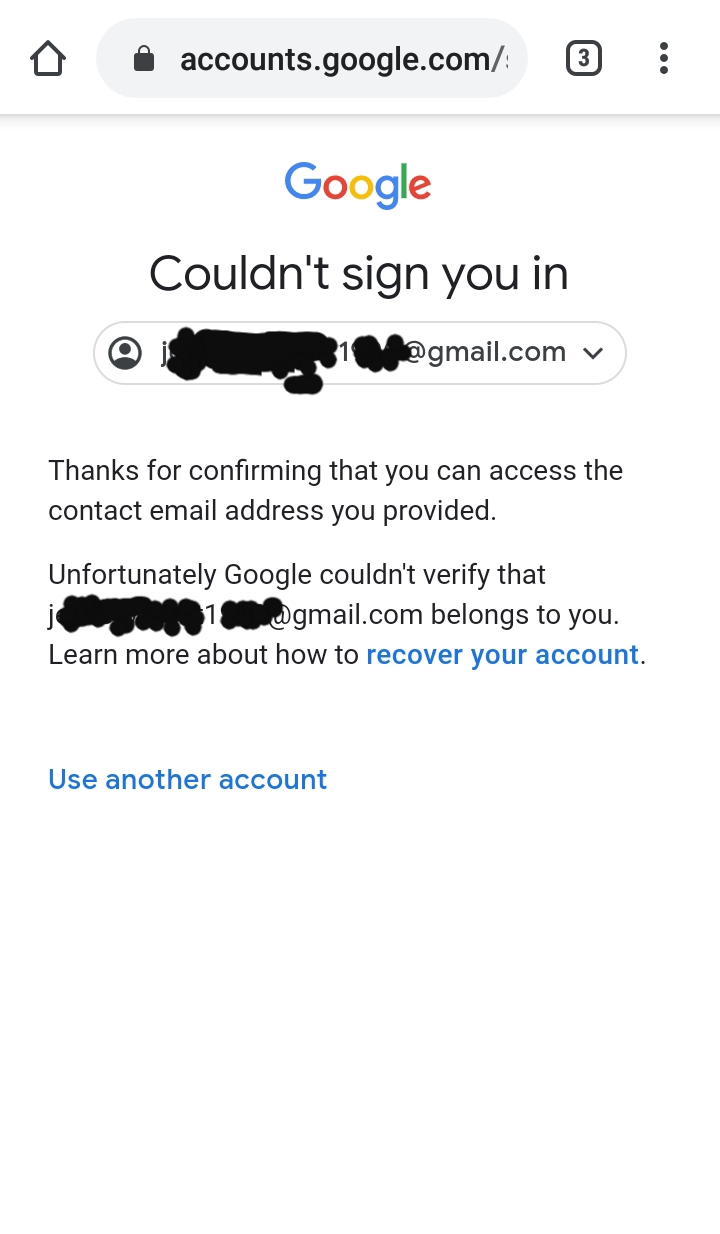The screenshot depicts a mobile phone displaying a webpage from accounts.google.com. At the top of the screen, there is a small box with the number "3," indicating that three tabs or windows are open. The Google logo, with its iconic multi-colored letters, is prominently displayed. Below the logo, there is a message in black text reading "Couldn't sign you in."

Partially obscured by black smudges, an email address is visible, showing only "one at gmail.com." Below this, a message thanks the user for confirming access to the contact email address provided, but it states that Google couldn't verify the ownership of the marked-out email address, which shows only a "J" followed by more black smudges. The message suggests learning more about account recovery with the phrase "learn more about how to," followed by a blue hyperlink text "recover your account."

At the bottom of the screen, another blue hyperlink text reads, "Use another account." The background of the webpage is white, and all text is in black. The browser's URL bar at the top shows a lock icon, indicating a secure connection, followed by the URL in a rounded box. To the right of the URL box, a small box with a "3" is present, and further to the right are three vertically aligned black dots, representing additional menu options. The entire interface has a clean and minimalistic design, adhering to Google's typical styling.